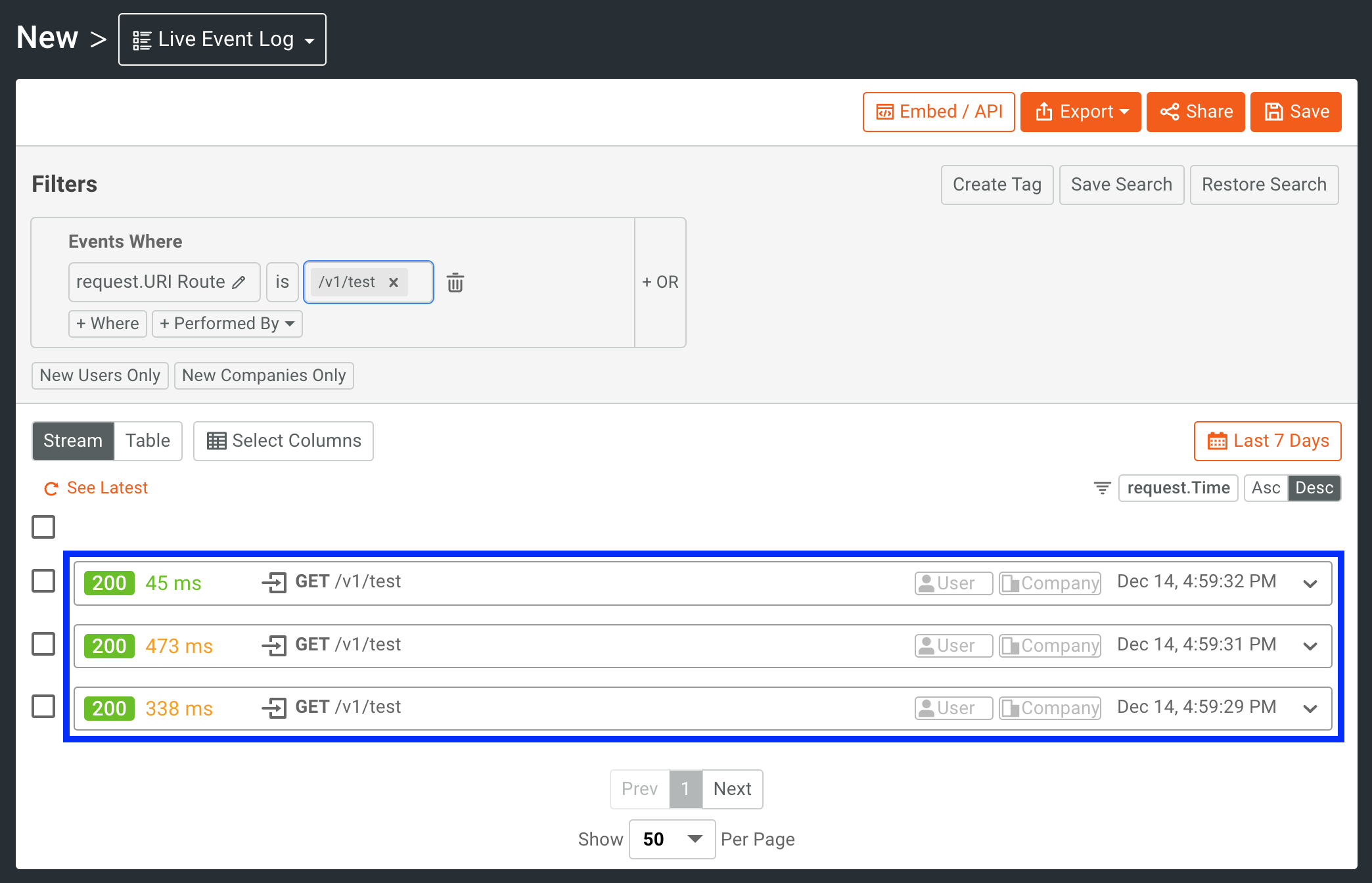This image is a screenshot of a web-based event log interface. At the very top of the page, there is a black banner labeled "NEW" alongside "LIVE EVENT LOG," indicating the real-time nature of the data being displayed. Below this header, the interface has a white background with various interactive elements.

Prominently featured at the upper section of the page, there are buttons in a vivid orangish-red or reddish-orange hue. These buttons are labeled "Embed/API," "Export," "Share," and "Save," providing users with options to interact with the event log data in different ways.

A calendar option, denoted by "Last 7 days," is highlighted with an orange border, enabling users to filter the logs within a specific timeframe. 

Lower on the page, there is a detailed event log consisting of several entries. Each entry is delineated within a royal blue rectangle, grouping them into a larger organized section. Specifically, three key entries are visible:

1. The first entry shows a status code "200" in a green rectangle, with a response time of "45 MS" for the endpoint "GET /v1/test."
2. The second entry also indicates a "200" status in a green rectangle, but with a longer response time of "473 MS."
3. The third entry again shows a "200" status in green, with a response time of "338 MS," highlighted in orange.

These entries provide detailed information on the status and performance of various API calls, making the interface a useful tool for developers and IT professionals monitoring live events.